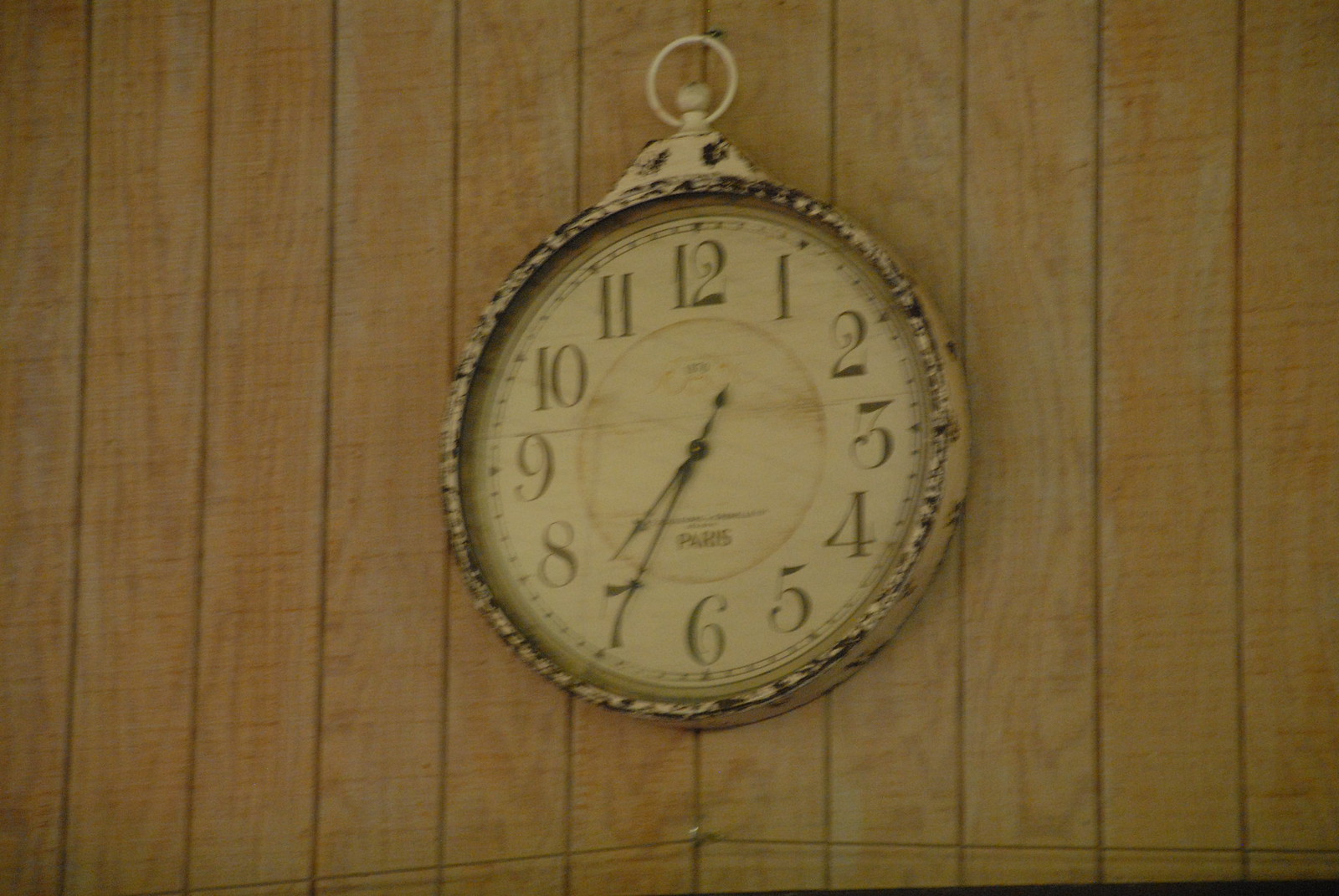The image showcases a wooden paneled wall with vertical planks running from top to bottom, creating a rustic backdrop. Centered on this wooden surface is a clock that closely resembles a giant pocket watch, complete with a loop at the top that mimics the feature used to attach a chain, enhancing its vintage appeal. The clock, however, is regular-sized and features classic clock numerals rendered in an old-time font, giving it an antique charm.

The bezel surrounding the clock face exhibits a distressed look, blending shades of gray, black, and likely silver, adding to the weathered, vintage aesthetic. The numerals on the clock face are a warm brown hue, contrasting softly against the background. The clock hands are strikingly slender and black, emphasizing the delicate nature of the timepiece. At the base of the clock face, just above the number six, there is a discernible word that appears to be "Paris," further hinting at a classic, nostalgic theme tied to a bygone era.